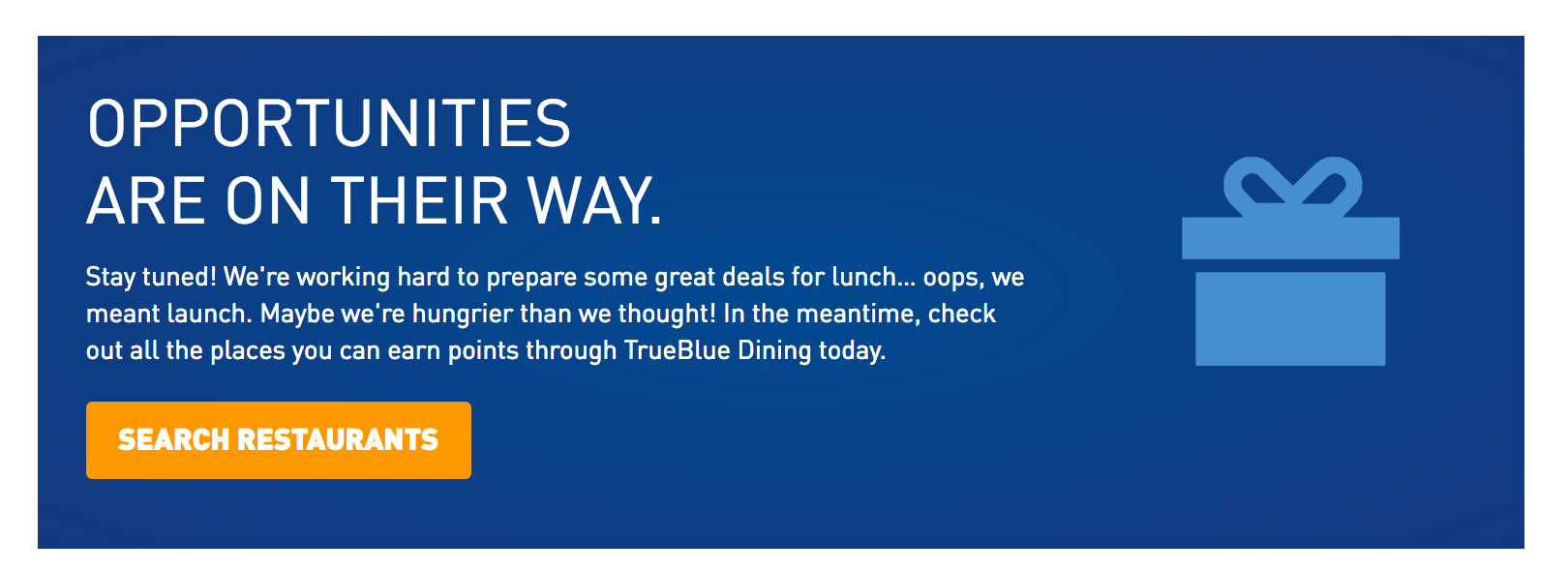A rectangular blue space is displayed, featuring a lighter blue gift box illustration on the right-hand side. The gift box is square with a rectangular top, resembling the lid, and is adorned with a ribbon outline. 

On the left side, aligned in larger, white text, it reads: "Opportunities are on the way." Below that, the message continues with: "Stay tuned. We're working hard to prepare some great deals for lunch. Oops, we meant launch. Maybe we're hungrier than we thought." Additionally, it encourages users to explore: "In the meantime, check out all the places you can earn points through TrueBlue Dining today."

Beneath this text, there is an orange rectangular box, which stands out with the white text inside stating: "Search Restaurants."